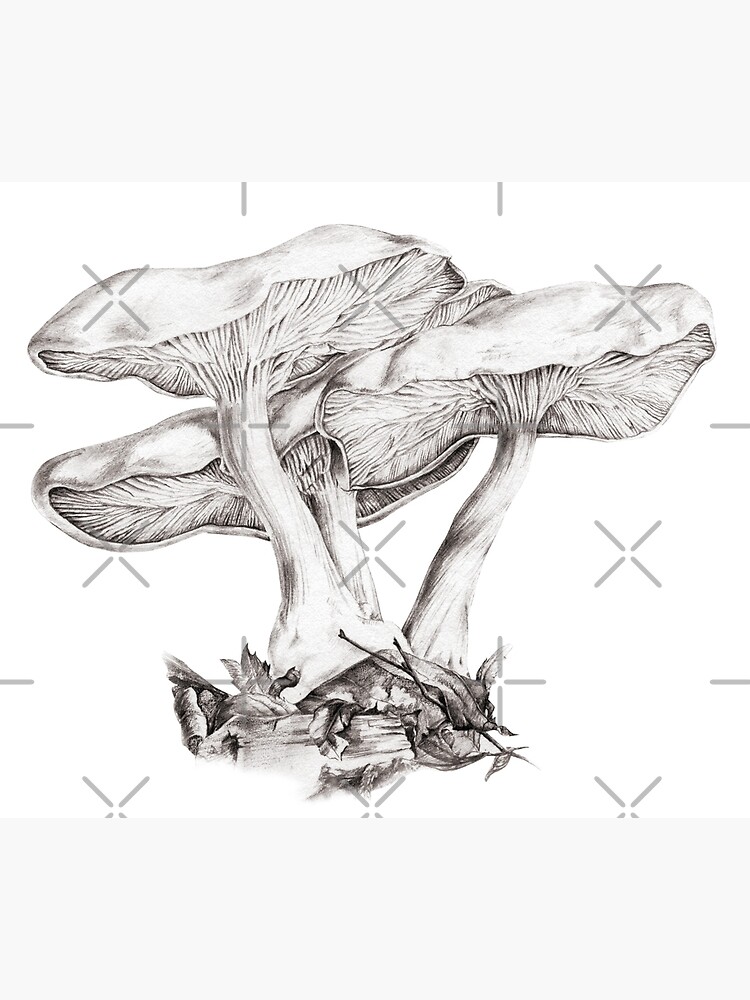This highly detailed black and white pencil drawing showcases three mushrooms of varying sizes—a short one, a medium one, and a tall one—each interconnected at their twisting stems. The mushrooms feature broad, flat caps that resemble little umbrellas, providing a whimsical image as if a cartoon mouse could sit underneath. The artist has meticulously shaded the drawing to highlight the textures, with visible lines on the underside of the caps and wavy, squiggly patterns. At the base, you can see elements of the ground such as grass, leaves, small chunks of wood, and other organic debris. The background is predominantly white, adorned with scattered gray X's and lines, which some appear to overlay the mushrooms, adding an interesting texture to the scene. Overall, it’s an exceptionally well-executed and intricate piece that captures the natural beauty and intricate detail of the mushrooms in their environment.